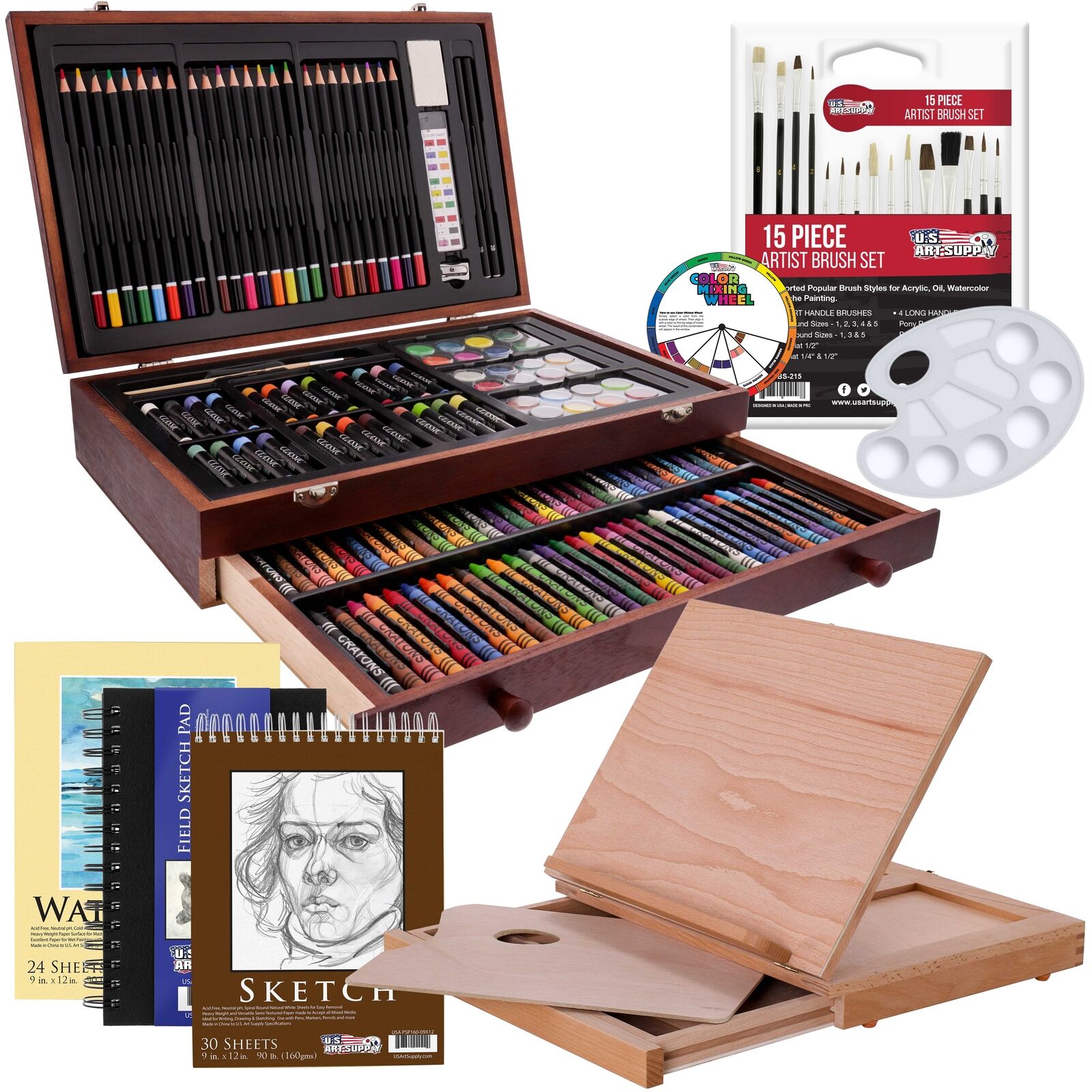The image depicts an expansive and meticulously organized artist's set, centered around an elegant wooden briefcase that serves as the focal point. The open briefcase reveals an array of art supplies: in its lid, a neat row of colored pencils spans various hues, including shades of blue, green, pink, and red, along with a pencil sharpener and erasers. The briefcase’s main compartment holds a versatile assortment of art tools, including adult crayon-like materials, a selection of paints—possibly acrylic or watercolor—and a drawer at the bottom with more crayons. 

To the upper right of the image, a prominently displayed 15-piece artist brush set in a white case claims attention, described with white lettering on red and black banners under the "U.S. Art Supply" brand. Adjacent to the brush set is a color wheel and a white palette for mixing paints, complete with a thumb hole for ease of use.

The bottom left section of the image features three distinct sketchbooks: a brown one prominently displaying a black and white sketch of a man, flanked by a yellow and a black sketchbook in the background. Finally, at the bottom right, there is another wooden structure resembling an easel, equipped with a drawer, suggesting it can be propped up to hold papers or canvases, with ample space for organizing various art supplies. This comprehensive art kit is designed to cater to a wide range of creative endeavors, from sketching to painting.